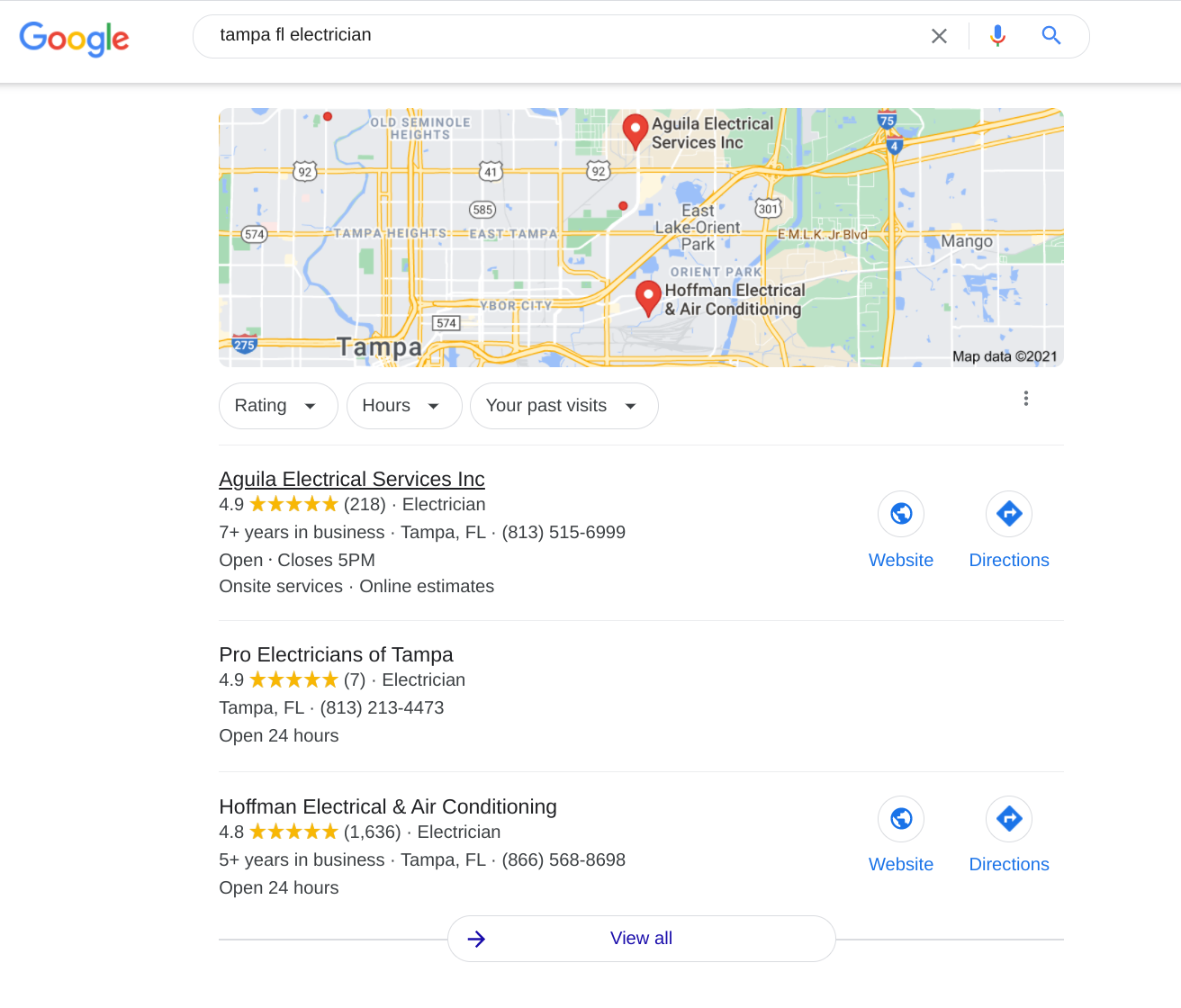The image is a cropped screenshot of a Google desktop search page displaying results for "Tampa Florida electrician." The background is predominantly white. At the top left, the Google logo is prominently displayed, followed by a long search bar to the right. Within the search bar, the text "Tampa Florida electrician" is typed in small black font. Adjacent to the text on the right, you see an 'X' icon to clear the search, a microphone icon for voice search, and a magnifying glass icon to initiate the search.

Below the search bar, centered on the page, is a large rectangular map featuring pin drops indicating various electrician locations within Tampa. Underneath the map, there are three drop-down boxes labeled "Rating," "Hours," and "Your past visits."

Further down, the search results are listed vertically. The first result is for "Agila Electrical Services Inc." The name is bold and underlined. Below it, the company has a 4.9-star rating from 218 reviews and is categorized as an electrician. It mentions that the business has been operating for over seven years in Tampa, Florida, and provides a phone number. The business hours indicate it is currently open and will close at 5 p.m. Additional services offered include on-site services and online estimates. To the right of this listing are two icons: a globe icon labeled "Website" in small blue letters, and an arrow pointing right, with "Directions" written below it.

The second search result is for "Pro Electricians of Tampa," followed by the third result for "Hoffman Electrical and Air Conditioning." At the very bottom of the screenshot, centered, is a "View All" button displayed in light blue.